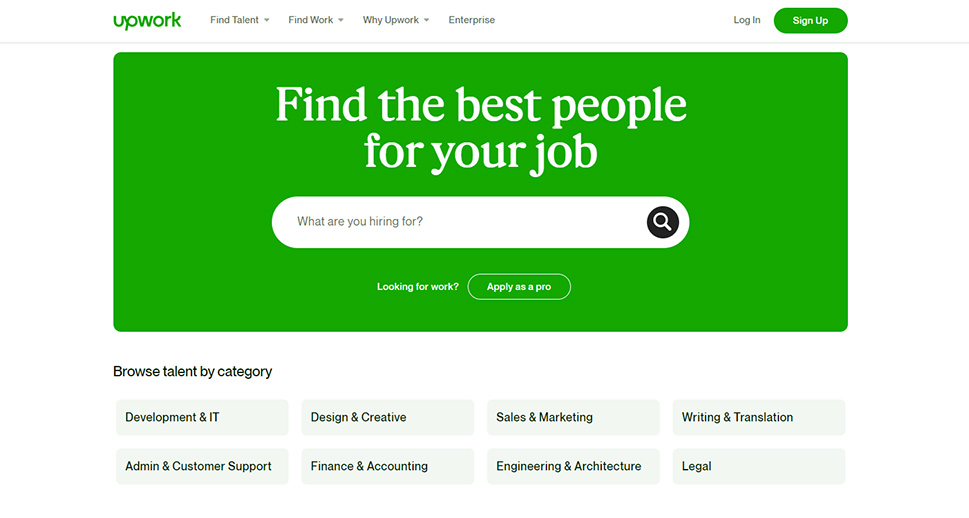The image displays a screenshot of an Upwork website page, characterized by a predominantly white background accented with green elements. At the top of the page, the word "Upwork" is prominently displayed in green. Adjacent to the logo are menu options labeled "Find Talent," "Find Work," "Why Upwork," and "Enterprise." Moving further to the right, there are buttons for logging in and signing up, with the "Sign Up" button highlighted in green.

Central to the page is a large green rectangular section containing the text: "Find the Best People for Your Job." Below this text, a search bar prompts users with the question, "What Are You Hiring For?" accompanied by a magnifying glass icon for initiating the search.

Beneath the green banner, there is a prompt "Looking for Work?" followed by a green button labeled "Apply as a Pro." Further down, the page lists various talent categories: Development and IT, Design and Creative, Sales and Marketing, Writing and Translation, Admin and Customer Support, Finance and Accounting, Engineering and Architecture, and Legal.

Overall, the webpage for Upwork presents a clean, straightforward design with a white and green aesthetic, focusing on usability and ease of navigation.